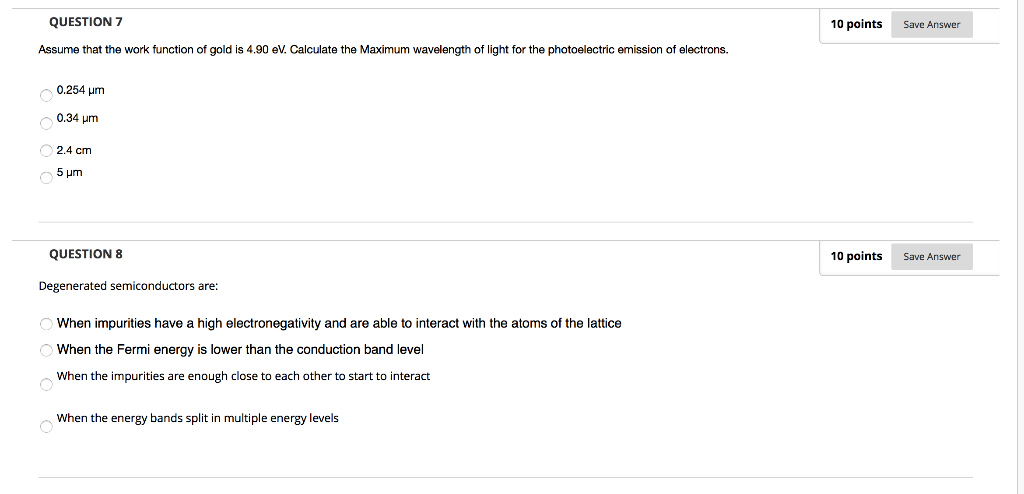In this image, set against a pristine white background, we observe a screenshot featuring black text situated below a light gray horizontal line. The highlighted content is for "Question 7," which asks: "Assume that the work function of gold is 4.90 eV. Calculate the maximum wavelength of light for the photoelectric emission of electrons." Positioned in the upper right corner, the text "10 points" and "save answer" are clearly visible. The provided multiple-choice answers for this question are: 0.254, 0.34, 2.4, and 5.

Two narrow gray lines demarcate the end of Question 7, leading into the bold, black text for "Question 8." This question states: "Degenerated semitic conductors are," followed by four potential answers: 

1. When impurities have a high electronegativity and are able to interact with the atoms of the lattice.
2. When the Fermi energy is lower than the conduction band level.
3. When the impurities are close enough to each other to start interacting.
4. When the energy bands split into multiple energy levels.

The upper right corner also indicates "10 points for the answer."